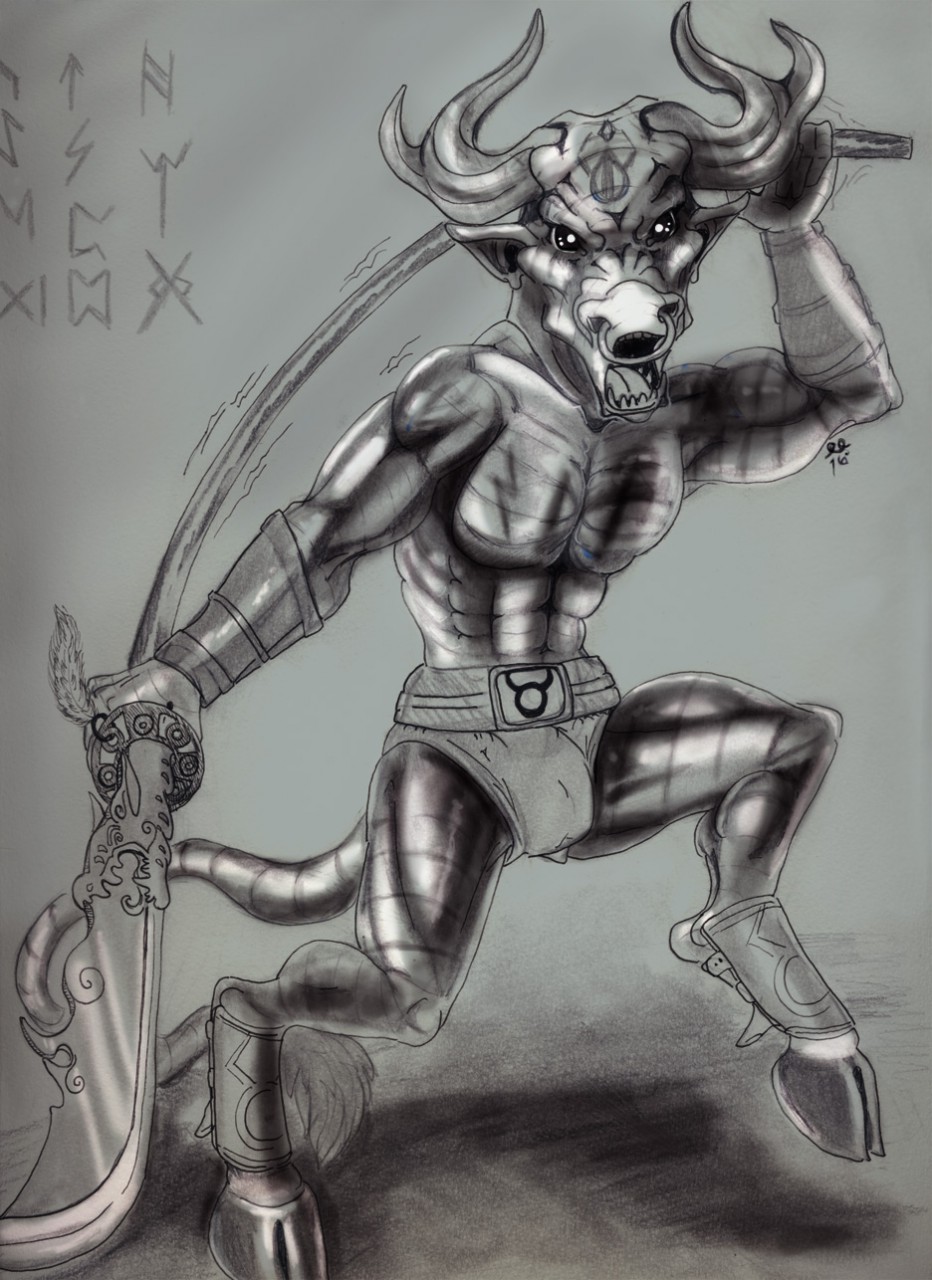The image depicts a hand-drawn, black-and-white pencil sketch of a menacing, anthropomorphic creature that blends human and ox-like features. The creature sports the horned head of a bull, which emanates a terrifying, almost demonic presence with fiery horns and a fiercely expressive face. Its muscular, chiseled physique is meticulously shaded in different tones of gray, emphasizing the artist's skill in creating depth and texture.

Standing on two legs, the creature exhibits hooves instead of human feet, adding to its otherworldly appearance. It wields a massive, jagged sword, which features a dragon-like design near the handle and evokes a sense of violent power. The creature also wears a loincloth or minimal underwear, secured by a belt that prominently displays the Taurus astrological symbol, further accentuating its mythical essence.

The background of the image is a gradient of light to dark gray, transitioning especially in the top left-hand corner where mysterious, archaic symbols or markings are visible. These symbols, scattered across both the background and the creature’s body, add an enigmatic and ancient aura to the overall composition. Shadows are skillfully depicted on the ground, accentuating the creature’s imposing stance—one hoof planted firmly on the ground, while the other is raised as if in mid-stomp.